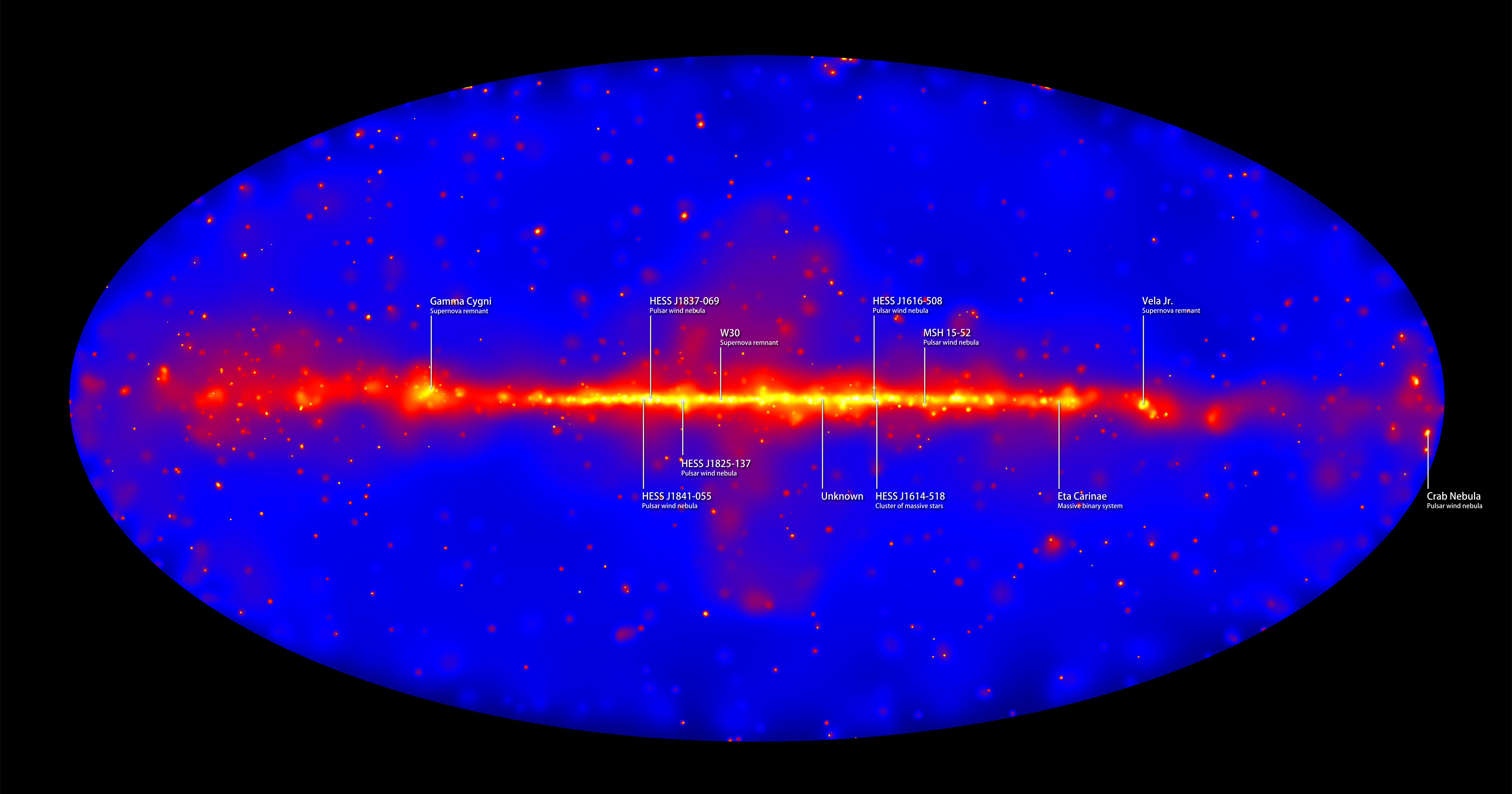This image depicts a detailed star map or astronomical composite. It features a deep blue oval set against a black background, suggesting a view of the night sky captured perhaps using UV or infrared filters. The oval itself, which is approximately twice as wide as it is tall, is dark fluorescent blue. A vibrant streak of red, orange, and bright yellow cuts horizontally through the center of the oval, signifying either a heated region such as a galaxy or interstellar gas. Numerous white lines emanate from this colorful streak, pointing to various locations and labeling them with names like Gamma, Sigma, Eta Carinae, and multiple Hess designated points (e.g., Hess J116, Hess J1614). These points are likely representative of stars, supernovas, or massive binary systems. Scattered across the image, predominantly within the oval, are many small red dots, adding to the impression of a densely mapped celestial region.